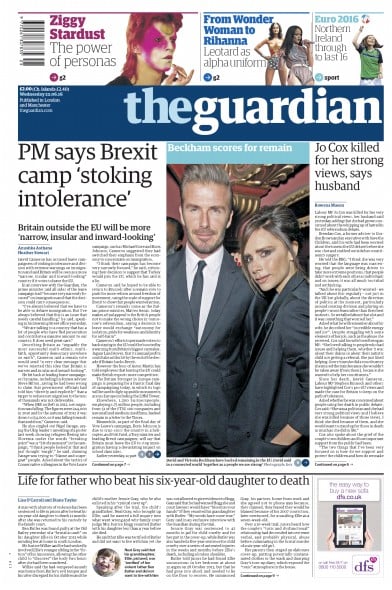A complex collage of images and text, this picture features multiple layers and themes. The central image appears to be a digital tablet held by a young girl, displaying content that seems to involve swiping. To the left of the tablet, the background intertwines various captions and articles, including a blurry yet prominent headline about Jo Cox, with a brief note on her husband's comments about her strong views. Further down, an image shows David Beckham in a sharp suit, accompanied by a woman also dressed formally, both facing the camera. Another segment of the image includes a cryptic mention of Brexit by Puma, hinting at the potential for continued intolerance. Additional text snippets seem to contain references and numbers that are challenging to interpret. Finally, a barcode is clearly visible at the top, seemingly linking or categorizing the collected content. The overall scene is disjointed yet richly detailed, offering a snapshot of various cultural and political narratives intersected by modern technology.